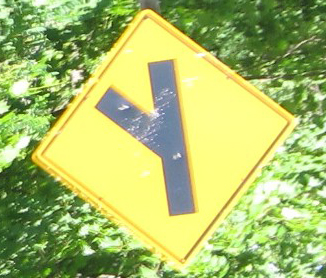This image captures a bright and sunny day in a rural area, featuring abundant green foliage from trees in the background. At the forefront stands a yellow, diamond-shaped road sign with a thin black border. The sign itself illustrates a black Y-shaped road, indicating a branching path ahead. The small square photo effectively conveys the serene and lush environment, emphasizing the sign's importance for navigating the rural setting.